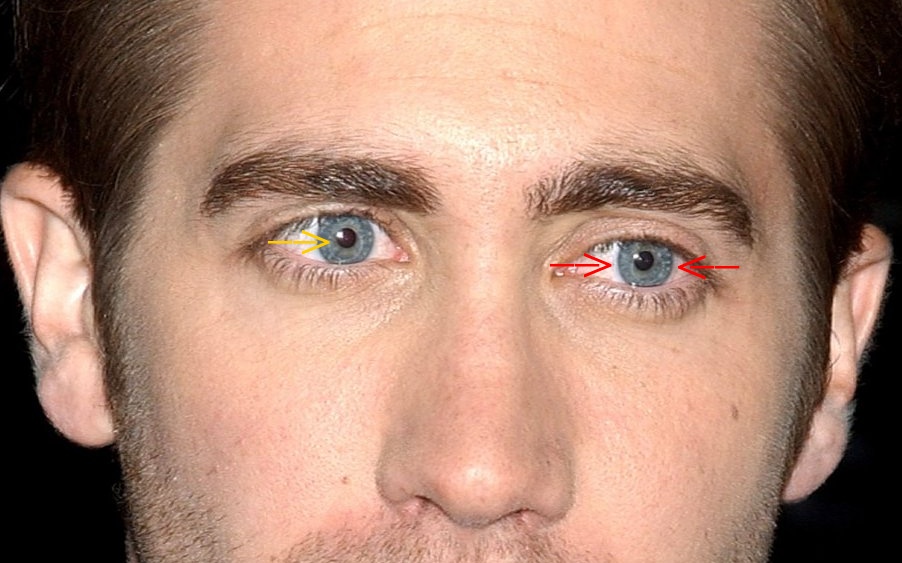A close-up photograph of a white man's face, featuring dark brown hair combed back with sideburns extending down before his ears, emphasizes his eyes against a black background. The image captures him from the middle of his forehead to below his nose, revealing his somewhat bushy eyebrows and unshaven look, with about one or two days' worth of stubble. His captivating gray eyes, slightly glancing to the left, are highlighted with added annotations: the left eye (on the right side of the picture) features two red arrows pointing at the iris, while the right eye (left side of the picture) has a single yellow arrow targeting the black pupil. This detailed editing draws attention to the intriguing colors and features of his eyes.